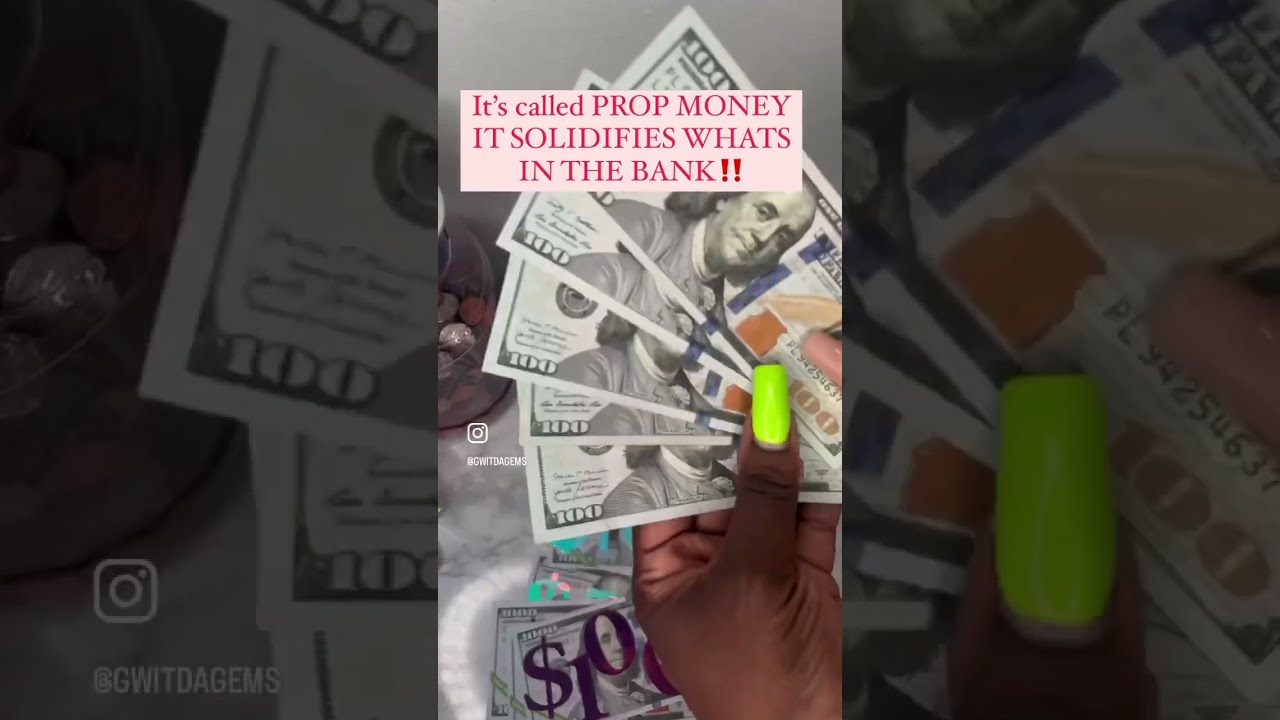In this promotional video still, the main focus is on a dark-skinned woman with bright lime green long fingernails, holding five brand-new $100 bills fanned out in her hand. The bills are detailed with a blue security strip and an orange or yellowish "100" in the corner. The background is a grey, blocked-out version of the same image, positioned in darker tones with an enlarged portion. Additional money is visible on the table in front of her and in the background, giving the impression of abundance. The top of the image features red text in a white box that reads, "It's called Prop Money. It solidifies what's in the bank!" On the left side of the image, there's an Instagram icon with the handle "@G-W-I-T-D-A-G-E-M-S," rendered in white over the icon. The overall setting appears to be indoors, likely her home, and the style is photographic representationalism.